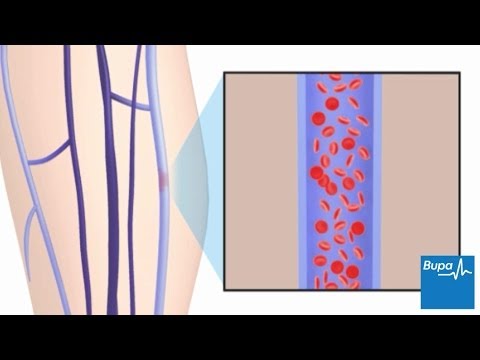The image depicts a detailed medical illustration focusing on a section of a vein, likely in the leg or arm, to highlight a potential blockage or thickening of the artery. The illustration features a prominent, vertical purple tube filled with numerous red blood cells, appearing like three-dimensional red disks. The purple tube is bordered by light lavender stripes on both sides, all set within a beige square with a black border. On the left side of the image, a transparent view of a limb shows interconnected dark blue and light blue veins. A zoomed-in section to the right of the limb provides a close-up of the vein, illustrating the flow of blood cells within it. The image is framed by black bars at the top and bottom, with a blue logo containing the word "Bupa" and a white EKG line situated in the lower right-hand corner. The primary intention of this detailed anatomical diagram is to visually explain blood flow through the arteries and veins.